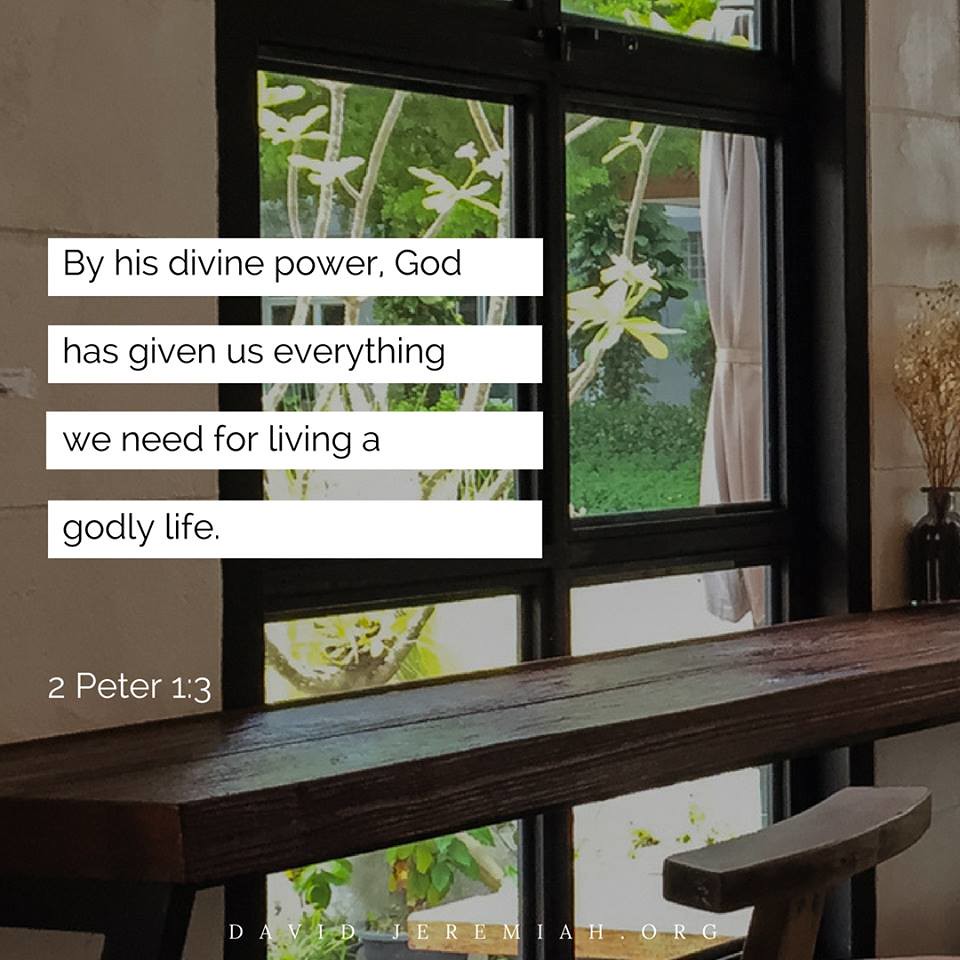The color photograph, commonly styled as a meme or inspirational poster, features a cozy indoor sitting area with a prominent large wooden bar made from a substantial piece of natural wood and a wooden bar stool. This setting is illuminated by a tall window with a black frame that offers a scenic view of a vibrant garden featuring plants, trees, and a small house to the right. The room's walls are made of white stone, enhancing the rustic charm of the space.

In the background, atop the wooden bar, sits a small vase filled with dried wheat, adding a touch of rustic elegance. The window, a focal point of the image, allows ample natural light to flood the room, contributing to the serene atmosphere.

Overlaid on this serene image is motivational text divided into four white rectangles with black font, sequentially reading: "By his divine power," "God has given us everything," "we need for living," "a godly life." Below this scriptural message, it cites "2 Peter 1:3," and at the very bottom of the image, the website "davidjeremiah.org" is displayed, guiding readers to further spiritual resources.